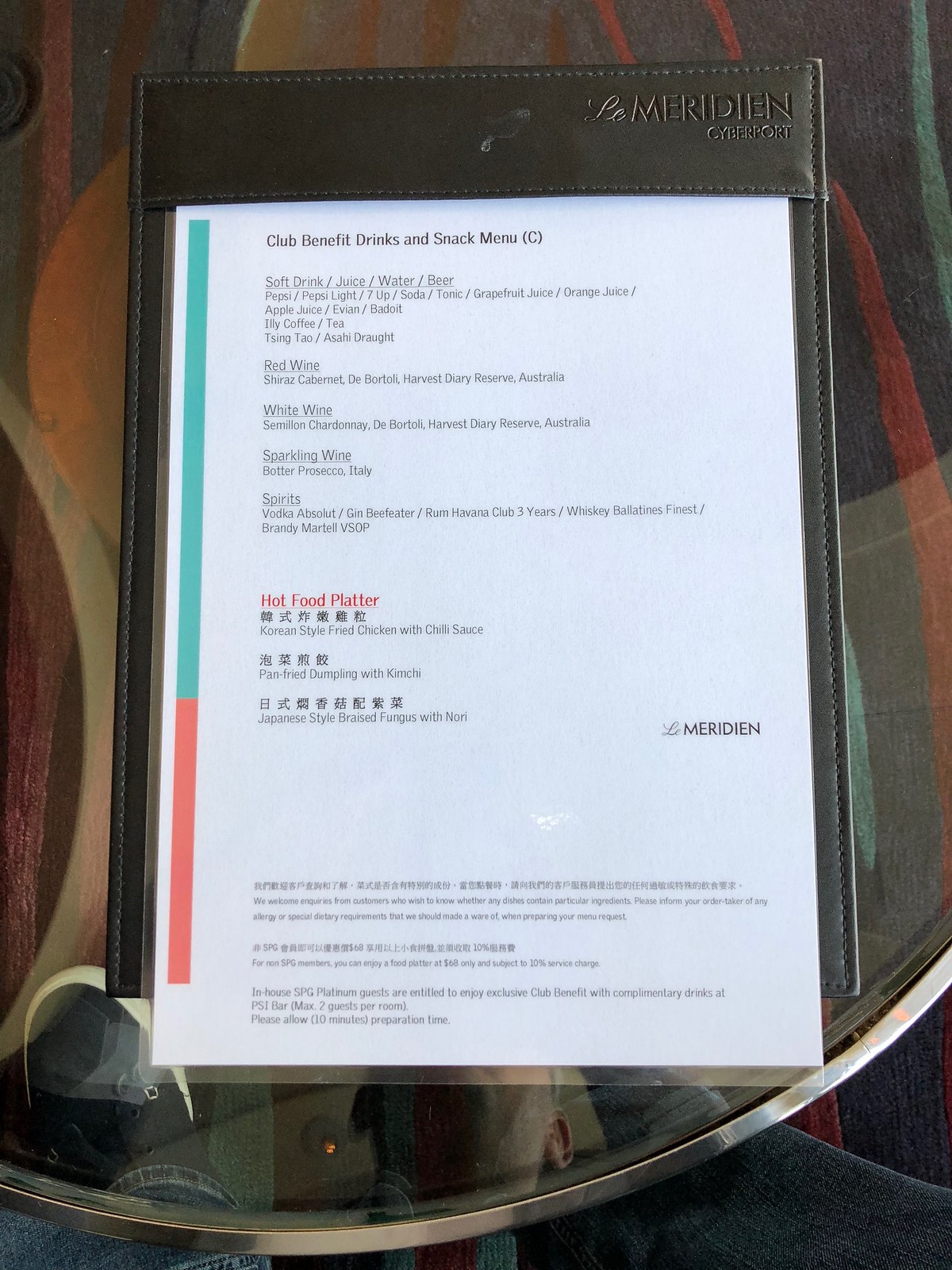This photo captures a menu at La Meridian displayed within a luxurious leather binder. The menu itself is encased in protective plastic sleeves and firmly secured within the binder. The main focus of the image is on the "Club Benefit Drinks and Snack Menu", prominently featuring a "Hot Food Platter". This platter lists three distinct items, each described in English with the corresponding Asian script above. The items include "Korean-Style Fried Chicken with Club Sauce" and a "Pan-Fried" dish, though the description is cut off.

The menu binder rests on a glass-top table, through which one can see the reflection of a gentleman. His attire consists of black tennis shoes and blue jeans, which are also visible under the transparent table.

In addition to the food offerings, the "Club Benefit Drinks" section boasts a variety of beverages, including soft drinks, juice, water, beer, coffee, tea, red wine, white wine, sparkling wine, and spirits.